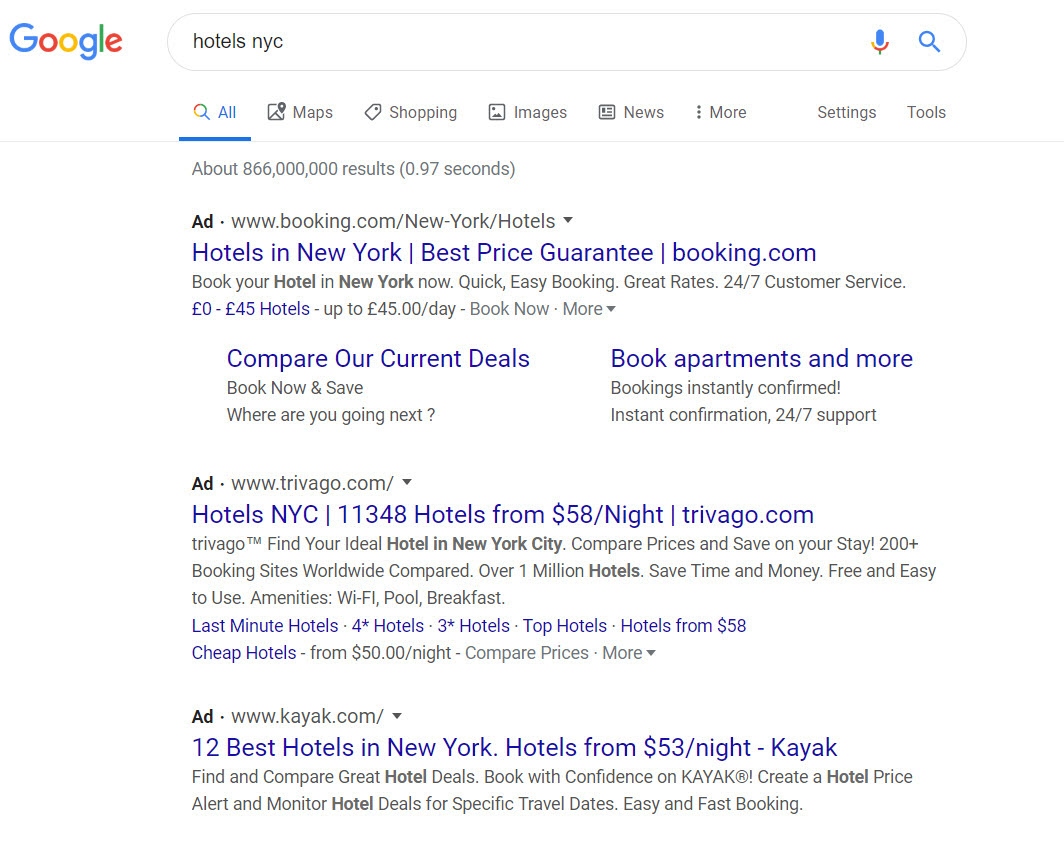This image is a screenshot of a Google search for "hotels NYC." The upper left corner prominently displays the colorful Google logo, followed by a search bar where the query "hotels NYC" is typed. Directly below the search bar, the user can see various clickable categories such as All, Maps, Shopping, Images, News, More, Settings, and Tools.

The main content of the screenshot features a series of advertisements for hotel booking sites. The top ad is from Booking.com, marked by blue text stating "Hotels in New York – Best Price Guarantee – Booking.com." Additional details mention that users can "Compare our current deals, book apartments, and more."

The second ad listed is from Trivago.com, which shows, "Hotels NYC – 11,348 hotels from $58 a night – Trivago.com," with some additional black text below it.

Lastly, there's an ad from Kayak.com, promoting "12 Best Hotels in New York – Hotels from $53 a night – Kayak." This ad also contains further descriptive black text underneath.

Each advertisement is presented in a block format, featuring prominent blue links and smaller black text descriptions designed to catch the user's attention.